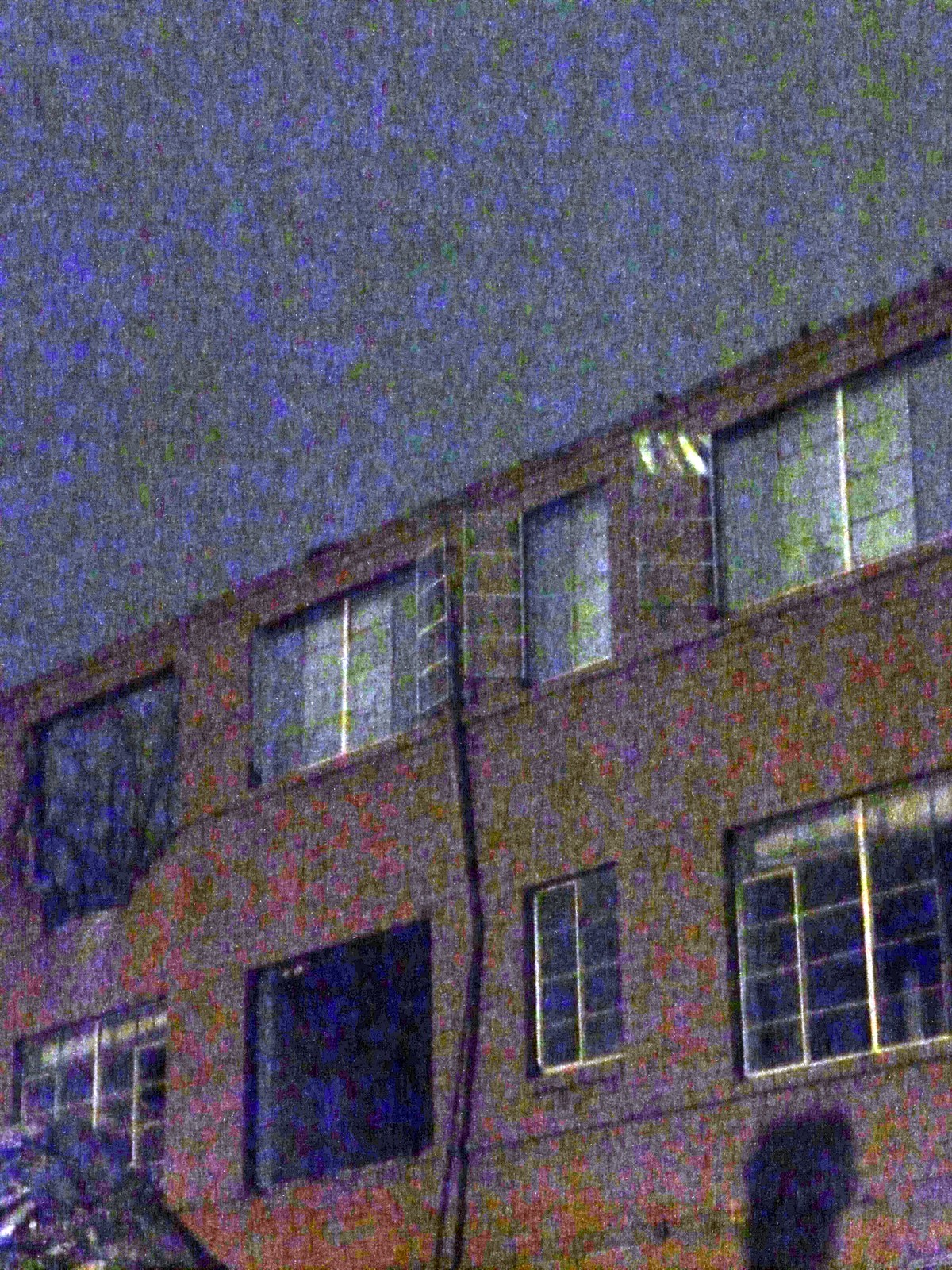A heavily blurred and oversaturated photograph captures the side façade of a brick building. The scene features four windows aligned at the top and three more on the ground level, with a central opening that resembles a doorway. Dominating the vertical axis, a thick cable runs from the base to the roof of the structure. In the lower right corner, the indistinct shadow of a human figure is faintly discernible. The left corner reveals a dark mound, which appears to be a pile of various materials, with colors blending into white, purple, beige, and green, resembling a small hill. The sky above is an eclectic mix of blue, green, and purple hues, adding to the surreal quality of the image. Notably, several windows are slightly ajar, hinting at activity within.